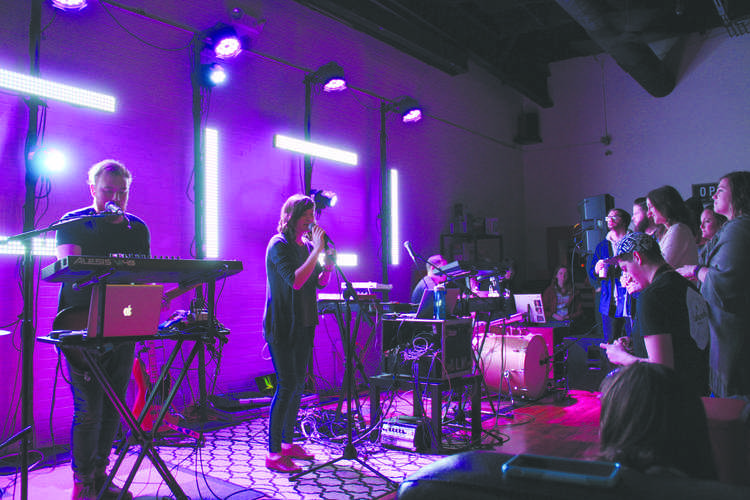In a small, intimate concert venue with a cozy carpeted floor and a vibrant pink wall as a backdrop, a band is performing. The stage is adorned with various musical instruments and cables, illuminated by purple LED lights and white stage lights. At the center of the stage, the lead vocalist passionately sings into a microphone. To the left, a man dressed in a black shirt plays the keyboard with a MacBook nearby, while to the right, a drummer keeps the rhythm. A small, captivated crowd of around 10 to 20 people is gathered on the right side, some watching intently and others occasionally glancing at their phones. The room is accented with visible ceiling pipes and assorted stage equipment, adding to the intimate, studio-like atmosphere.